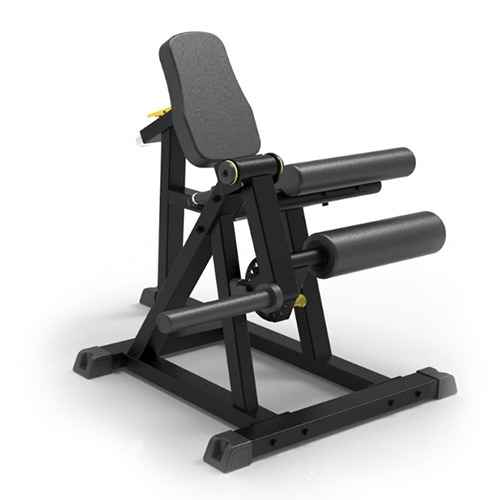Against a solid white background that occupies most of the space, the color photograph showcases a portrait-oriented image of a piece of gym exercise equipment designed for leg training. The equipment features a black, padded seat with a slanted backrest leaning toward the top left of the image. A vertical black post behind the backrest provides support, while a horizontal black rod covered in flexible black foam is positioned below the seat, intended for placement in front of the shins during leg lifts. The machine includes two cylindrical rollers at the front—the bottom roller being slightly larger than the top—contributing to the leg exercise mechanism. Adjacent to the equipment, there's a black bar with a long cylindrical extension and an attached rotating crank mechanism that presumably adjusts the intensity of the weights. The base of the equipment forms a rectangular structure with four intersecting black bars, providing stability. The photograph is detailed, clear, and realistic, accurately representing the exercise machine against its minimalist backdrop.